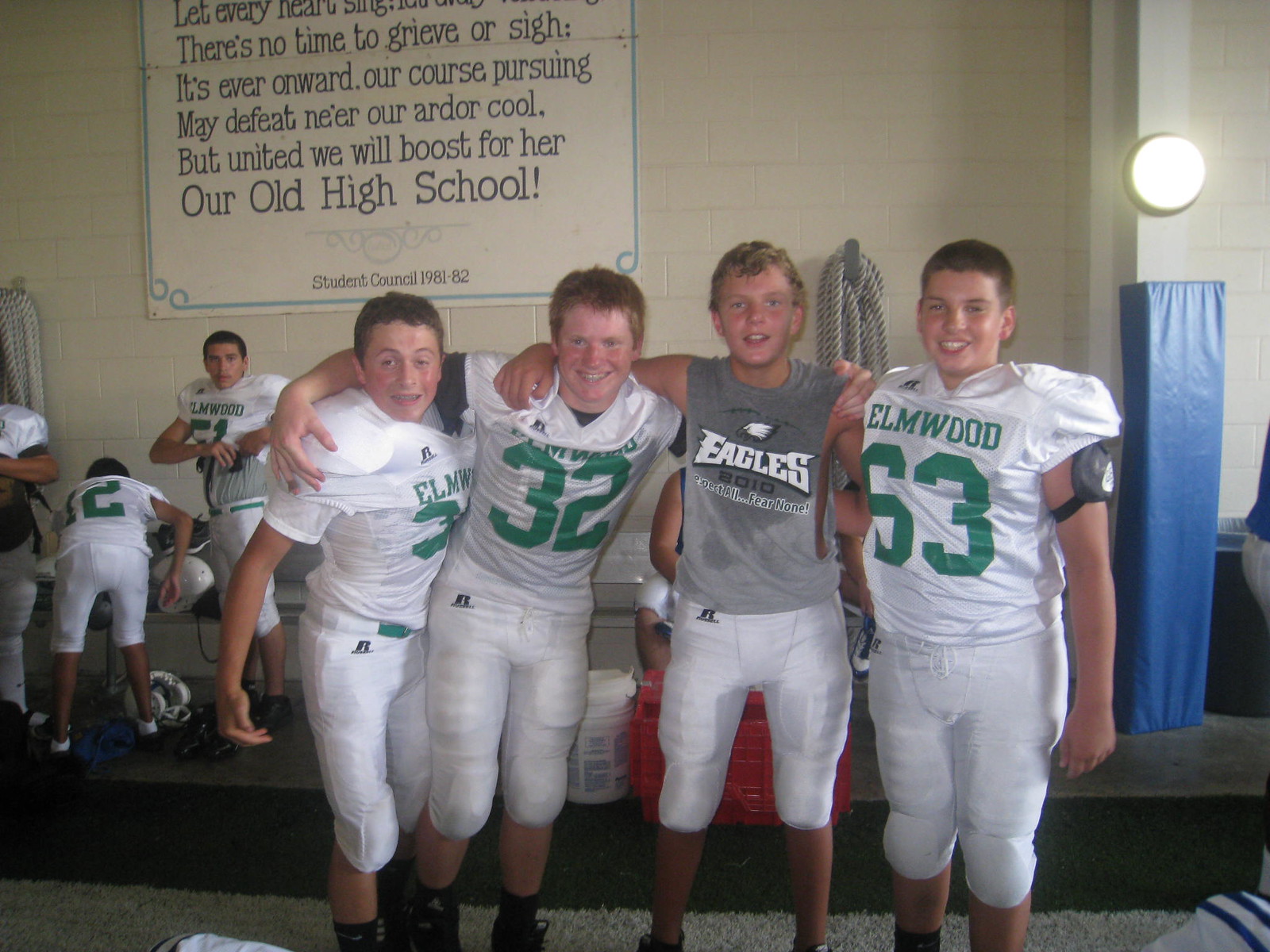This photograph captures a group of four high school boys posing together in their football uniforms inside a locker room. They stand with their arms over each other's shoulders, all smiles, wearing uniforms that feature white jerseys with green "Elmwood" text and player numbers, paired with white pants and black socks. The third boy is different, wearing only the football pants and a sleeveless gray t-shirt that says "Eagles." A background of activity is visible with other players in various stages of dressing or undressing for a game. Affixed to a concrete wall behind them is a large sign bearing a motivational statement: "There is no time to grieve or sigh, it's ever onward, our course pursuing; may defeat never cool our ardor, but united we will boost for her, our old high school. Student Council 1981-82." A thick rope is hooked onto the wall near the sign. The scene is set on beige and brown carpet, with a blue-and-white section of the wall and a bright white light adding to the vividness of the environment.